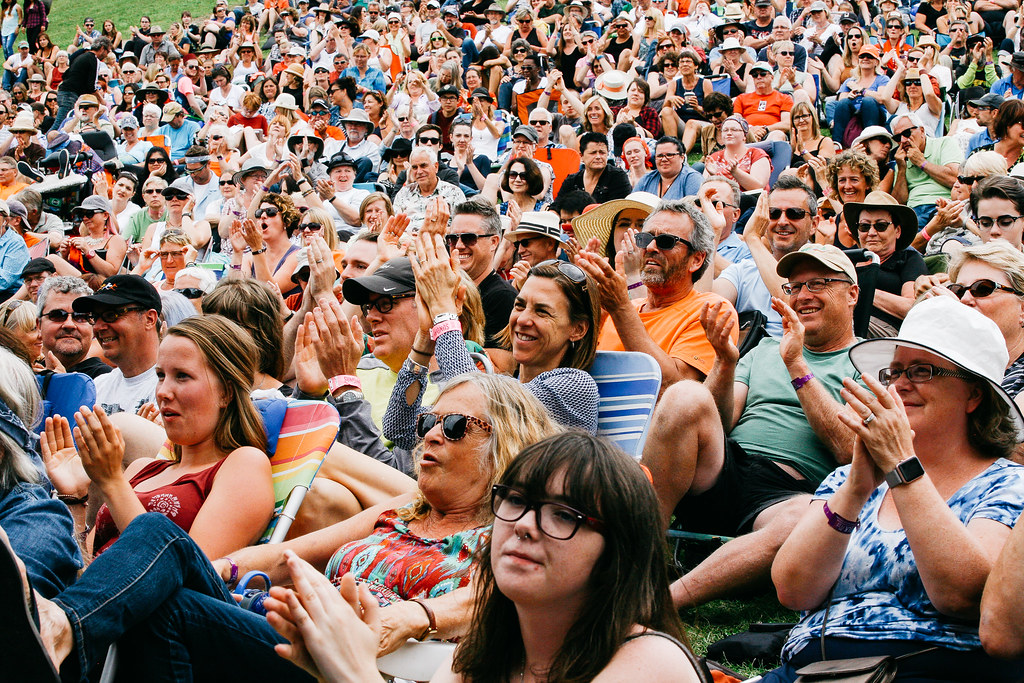This vibrant, full-color photograph captures a sprawling crowd of hundreds, composed primarily of Caucasian men and women of various ages, from teenagers to those in their 50s and 60s, seated closely together on a grassy lawn. It appears to be a warm, sunny day, given they are dressed in casual summer attire such as T-shirts, tank tops, jeans, and shorts, complemented by an array of hats and sunglasses. The attendees are sitting on an eclectic mix of personal lawn chairs, all facing forward towards an unseen focal point, likely enjoying a concert or a festival performance. Clapping and smiling, they radiate a joyful and engaged energy. The densely packed crowd, with individuals nearly shoulder to shoulder, evokes a lively and festive summer atmosphere, reminiscent of a 'Where's Waldo' scene teeming with vivid detail.